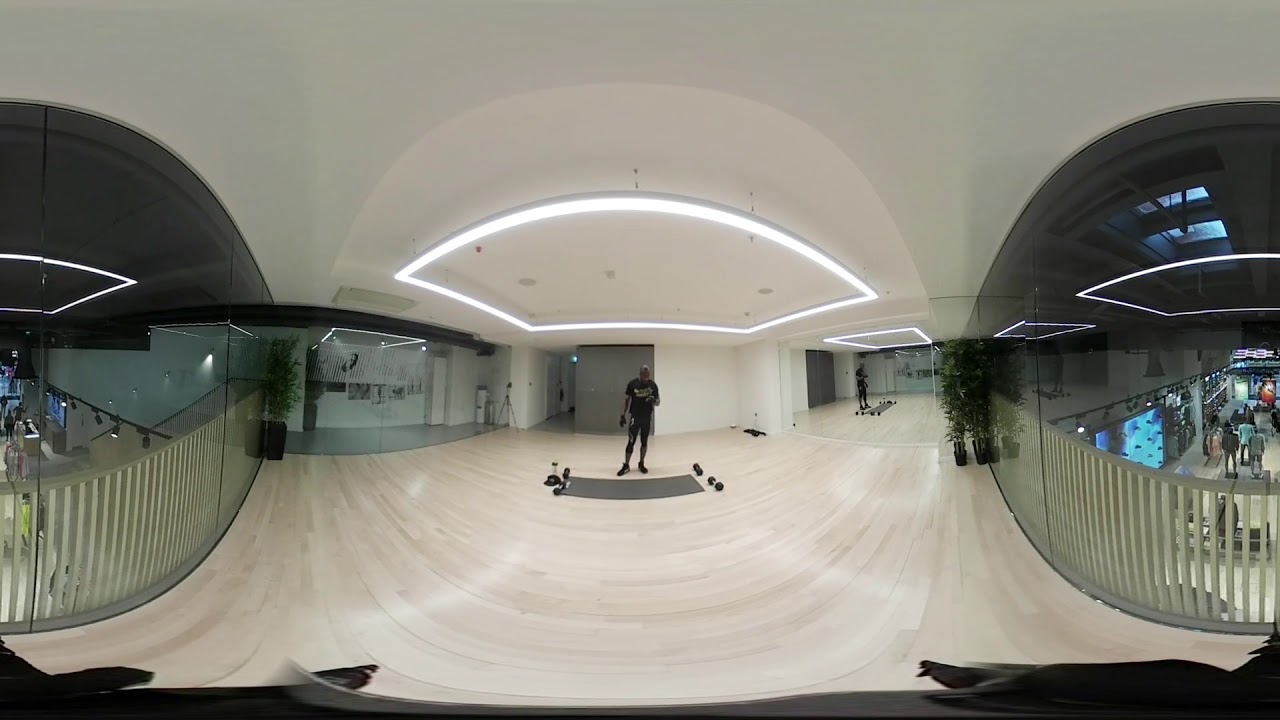A panoramic 360-degree photograph taken inside a fitness studio, situated in a mall. At the center of the image stands an African or African American man with dark brown skin, dressed in an all-black outfit including a black t-shirt and shoes. He is slightly leaning to the right, his feet pointed left and forward, and is looking down at a device in his hand with one arm bent at a right angle close to his body and the other by his side. In front of him lies a light gray rectangular mat with black dumbbells on either side. Above, the ceiling is white with a square light fixture and a sunroof visible on the right. The flooring underneath is a light beige or cream wood color, transitioning to gray near the mat.

The walls of the room are made of glass, offering views into an adjacent shopping area. On the right side, a large glass mirror reflects part of the fitness studio, while glass doors on the other side lead to a small area with a drinking fountain. Through the surrounding glass, the bustling environment of a mall can be seen, with shoppers, stores, and indoor walkways below, all illuminated by various lights. Additionally, a tripod or camera setup is noticeable in the background on the left side of the room. There is also a black hat with white writing on the ground near the man. White railings or posts are visible along the edges of the upper floor's perimeter, and the borders of the ceiling are lined with white spotlights, adding to the bright, airy atmosphere of the space.